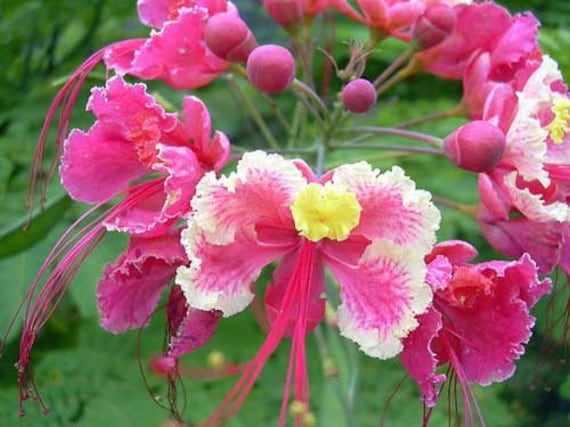The image captures a stunning flower bud at the center, accentuated by lush, green foliage in the blurred background. The primary focus is a single flower showcasing multiple fuchsia-colored floral petals that form a circular, pom-pom-like structure. Among the closed petals, there's a captivating bloom with petals edged in white, revealing a vibrant yellow center flower. Surrounding this central blossom are a few additional unopened bulbs and buds. The flowers exhibit a pattern as if they are rotating around a central stem, with three prominent buds and a fourth slightly apart, on the right. Some of the flowers display pinkish strands emerging from their centers, possibly part of the pollen structures, adding to the intricate detail of the composition. The overall aesthetic is harmonious, with the rich fuchsia, pink, and yellow hues standing out against the serene green backdrop.